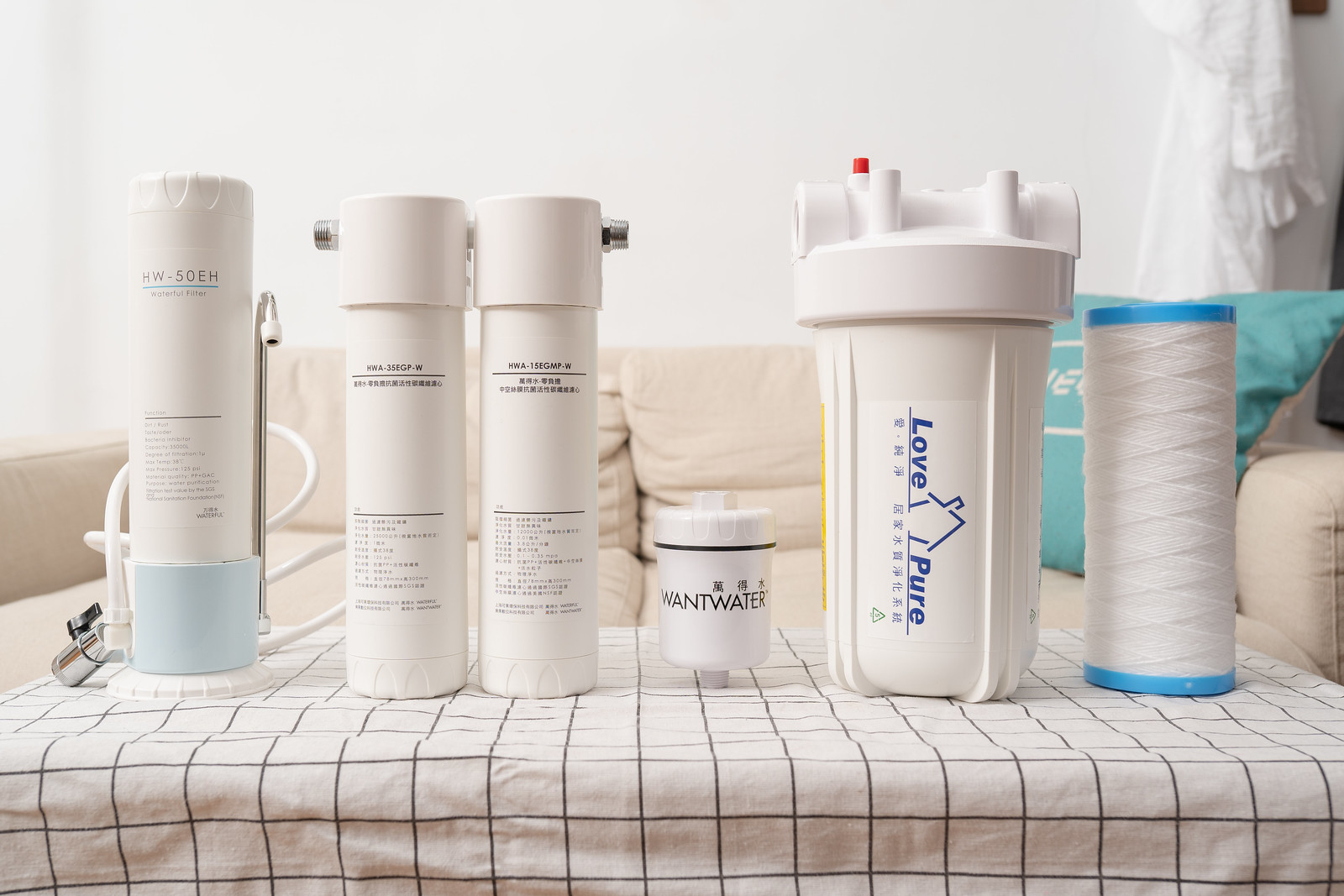This detailed photograph showcases a room with a plain white wall adorned by a hanging white bathrobe in the background. Central to the image is a white sofa displaying white cushions and a turquoise pillow positioned on its right side. In front of the sofa is a table draped with a towel or blanket characterized by a white and black grid pattern. On this table, various cylindrical hygiene products are meticulously arranged. Among them is a spool of white thread, and multiple white plastic containers featuring Chinese writing. One container bears the word "LOVE" and another "WATER," each inscribed in both English and Chinese. Additionally, there is a cylindrical device with a light green base and a chrome hose ending in an on/off valve. The table also hosts Q-tips and possibly other small bathroom items, completing the display of personal care products.